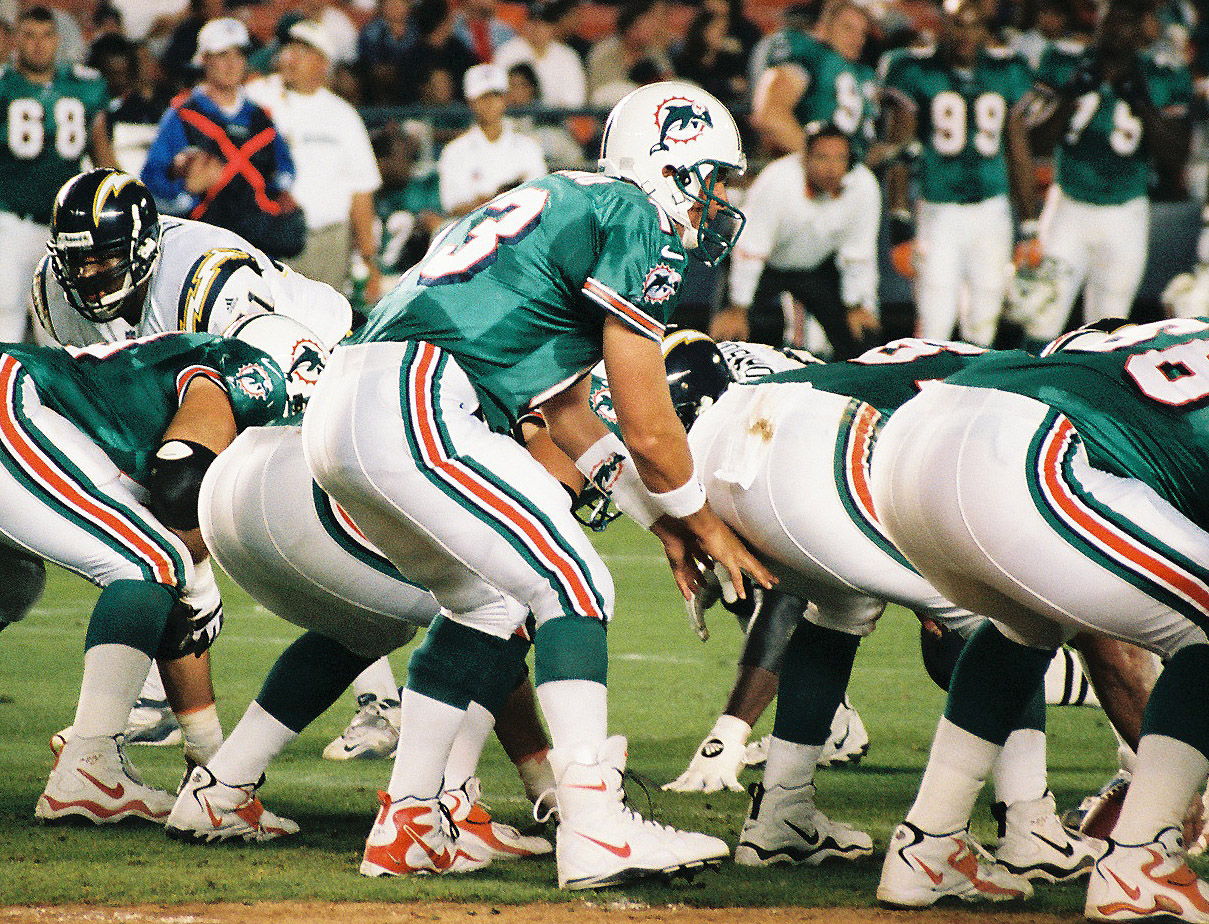The photograph captures a Miami Dolphins football game against the San Diego Chargers, focusing on a pivotal moment just before the play begins. At the center of the image, slightly left of the middle, stands quarterback Dan Marino, identifiable by his number three jersey and his white helmet adorned with the iconic green dolphin and red circle insignia. Marino is positioned under center, ready to receive the snap from his bent-over linemen, whose distinctive green and orange striped pants and white cleats with orange Nike checks are visible. The Dolphins' offensive line is prepared, with two linemen to Marino’s right and two to his left, their uniforms featuring green and orange accents along with wristbands that showcase the team logo encircled in orange. Facing them are members of the Chargers’ defensive line, partially seen towards the left and just to the right of Marino's extended arm.

In the background, beyond the players, the sideline is visible with more Dolphins personnel, including number 68 on the far left, a ball boy, coaches, and additional players. The stands, filled with spectators, form a blurry backdrop in the upper portion of the image, emphasizing the in-focus action at the line of scrimmage. The overall composition is angled, with the Dolphins' offense facing right and slightly away from the camera, creating a dynamic sense of anticipation just moments before the play unfolds.